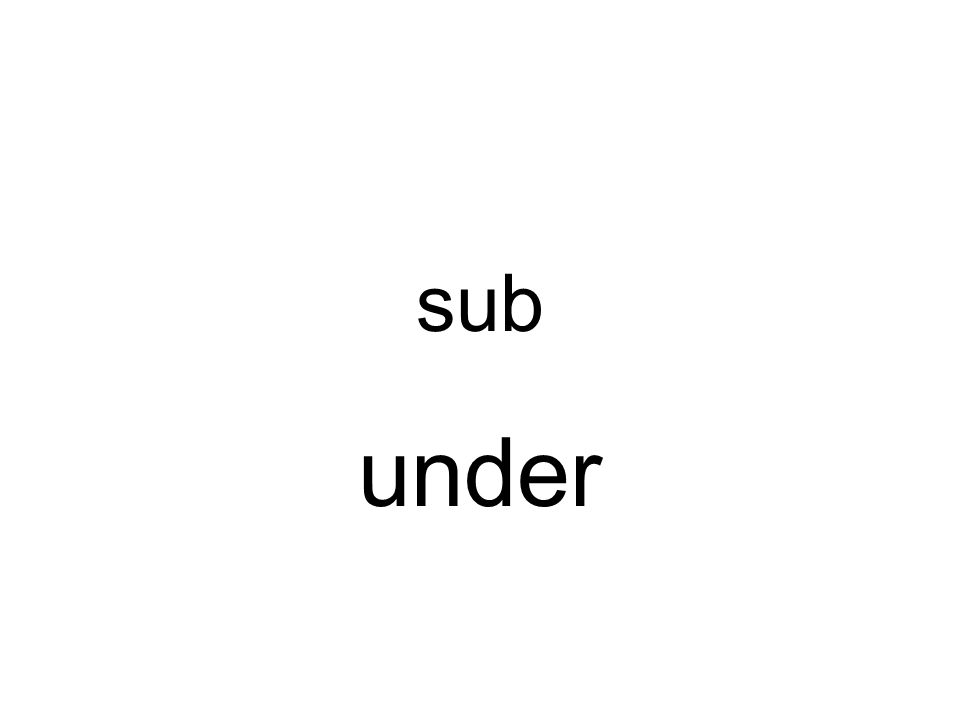The image features a minimalist design with two words centered on a solid white background. The top word, "sub," is rendered in all lowercase letters and appears slightly smaller in font size compared to the word below it. Positioned a few spaces down, the word "under," also in lowercase, is larger and draws more attention. Both words are in black text, with ample spacing between them, creating a clear visual hierarchy. The font resembles a clean, sans-serif style, akin to Helvetica. The simplicity and lack of visual elements suggest versatile applications, such as educational materials, presentation slides, or even potential artwork for album covers.